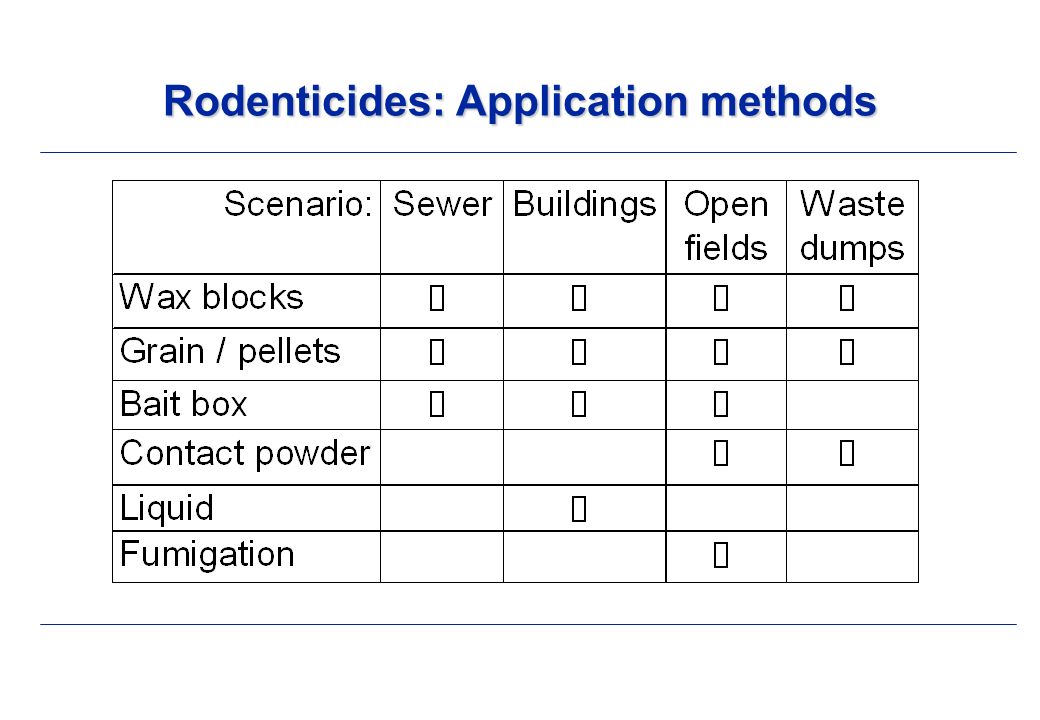The image features a chart detailing various application methods for rodenticides, titled "Rodenticides: Application Methods" in bold blue font at the top center. Below the title is a thin blue horizontal line, followed by a neatly organized grid with black lines, set against a plain white background. The chart consists of five columns and seven rows. The top row lists the columns: "Scenario," "Sewer," "Buildings," "Open Fields," and "Waste Dumps." The first column from the top to the bottom reads: "Wax Blocks," "Grain/Pellets," "Bait Box," "Contact Powder," "Liquid," and "Fumigation." 

For "Wax Blocks" and "Grain/Pellets," all cells corresponding to "Sewer," "Buildings," "Open Fields," and "Waste Dumps" are marked, indicating they are applicable in these scenarios. In the "Bait Box" row, all cells except "Waste Dumps" are marked. The "Contact Powder" row has marks under "Open Fields" and "Waste Dumps," with no marks for "Sewer" and "Buildings." For "Liquid," only the "Buildings" cell is marked. Lastly, "Fumigation" is marked only under "Open Fields." Another thin blue line runs horizontally at the bottom of the chart.